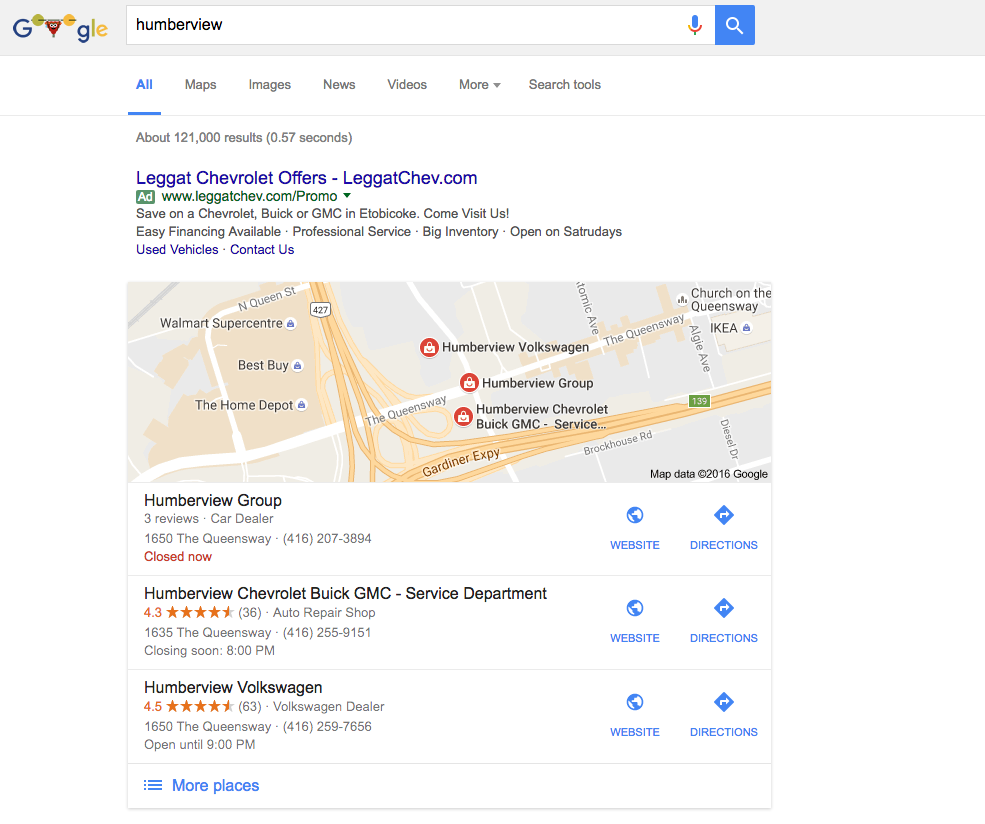The image features a Google search results page for the query "Humberview." At the top, the iconic blue Google "G" logo is prominently displayed within a gray navigation bar across the screen. The full colorful Google logo includes a blue "G," yellow "o," red "o," blue "g," green "l," and yellow "e."

Below the navigation bar is a search bar containing the text "Humberview." The page’s navigation tabs follow, including "All," "Maps," "Images," "News," "Videos," "More," and "Search tools," with "All" highlighted in blue and underlined, signifying it is the currently active tab.

The search results indicate approximately 121,000 results. The first result displays "Leggett Chevrolet offers" with the URL "www.LeggettChev.com" labeled as a green ad, followed by "Slash promo" and an arrow pointing downward.

A map is shown further down, highlighting different locations including Humberview Volkswagen, Humberview Group, and Humberview Chevrolet Buick GMC Service, each marked with red circles and shopping bag icons. Humberview Chevrolet Buick GMC Service has a rating of 4.3 stars, while Humberview Volkswagen holds a 4.5-star rating. Both businesses have their website links and directions available in blue text.

A horizontal line delineates the map section from additional options, with three blue bars indicating "More places." At the bottom of the map, the text reads "Map data 2016 Google."